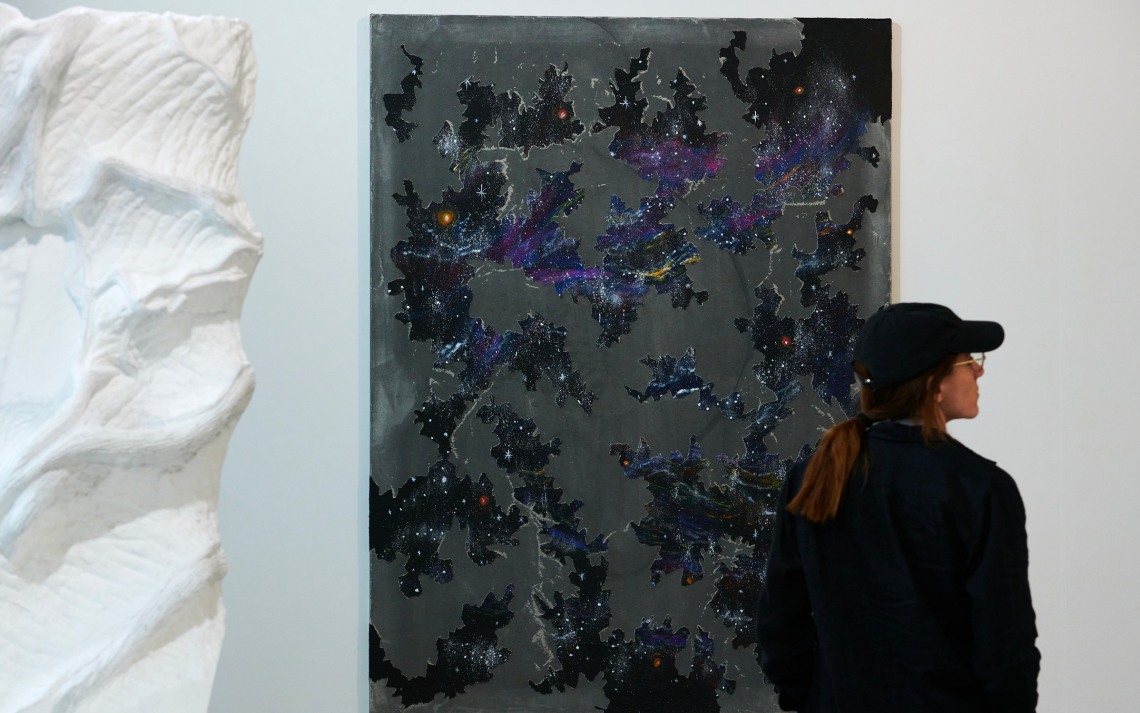The photograph portrays a woman standing in an art gallery, positioned in front of a large modern art piece dominating the center background. The artwork features a chaotic mix of colors resembling Rorschach test blots or an incomplete puzzle set against a gray and silver backdrop, evoking a nebula-like imagery with scattered white dots and star-like elements. The woman, standing near the right side of the frame with her back to the camera, slightly turns to her right, revealing a bit of her profile. She has a long ponytail tucked into a hat, is wearing glasses, and her outfit appears dark, possibly due to lighting. To the left of the central art piece, part of a white sculptural artwork is visible, seemingly ceramic, with folds and lines that hint at a classical or Egyptian influence. The overall scene strongly suggests the setting is an art museum or gallery.